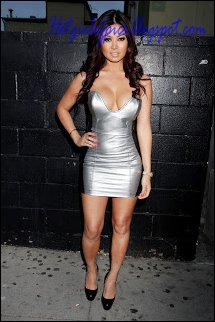This image is a small, vertically aligned photograph, approximately an inch and a half wide by two and a half inches high. It captures a full-body shot of a woman standing confidently on a gray speckled sidewalk, her right hand poised on her hip while her left hand rests by her side. She is posing in front of a black cinder block wall that is shorter than her, with another wall visible in the background, and a few indistinct black marks, possibly small leaves, scattered on the ground. 

The woman, who might be a model or an actress, is dressed in a form-fitting, strapless silver mini dress that reaches her upper thigh and accentuates her figure. Her long, wavy dark brown hair cascades over her shoulders. She is also wearing black heels, adding to her poised look. Above her head, purple or blue lettering can be seen, though it is difficult to decipher. It appears to be a website, potentially reading "hotgirlformegaspot.com". Despite the low readability, the last part, "dot com," suggests it is indeed an online address. The woman is smiling slightly, contributing to the overall confident and stylish demeanor conveyed in the photograph.